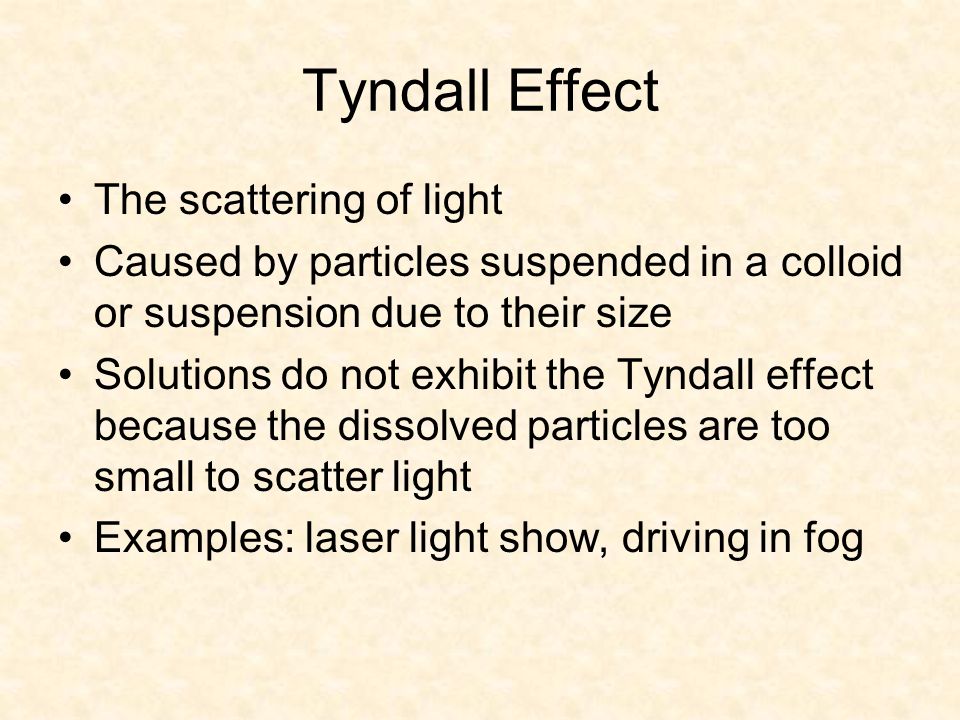The image appears to be a slide from a presentation, featuring a medium tan or beige tiled background. In large, bold black letters at the top center, it reads "Tyndall Effect." Below this heading are four bullet points, each spaced slightly apart and typed in black font. The bullet points delineate key aspects of the Tyndall Effect:

1. "The scattering of light."
2. "Caused by particles suspended in a colloid or suspension due to their size."
3. "Solutions do not exhibit the Tyndall Effect because the dissolved particles are too small to scatter light."
4. "Examples: laser light show, driving in fog."

The text is neatly formatted and centrally aligned, providing a clear and detailed explanation of the Tyndall Effect.